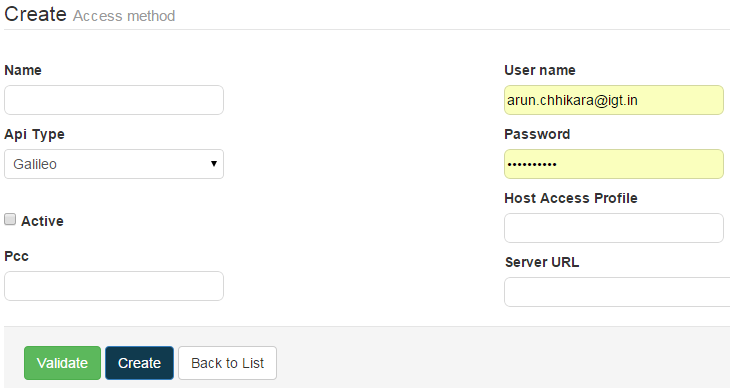This image displays the sign-in or registration section of a website against a white background. At the top left, the bold black text "Create" is prominently displayed, while "Access Method" is written in light gray to the right of it. A light gray line separates these titles from the form below. 

The form begins with a field labeled "Name," accompanied by a box for input. Below this is a drop-down box labeled "API Type," currently set to "Galileo." Following this is an option to check or uncheck a box labeled "Active." Further down, a field labeled "PCC" is provided with an input box next to it.

On the right side of the form, "Username" and "Password" fields are present, both containing entered information. Below these, there are fields labeled "Host Access Profile" and "Server URL," each accompanied by empty input boxes.

At the bottom left of the image, three buttons are visible: "Validate," "Create," and "Back to List."